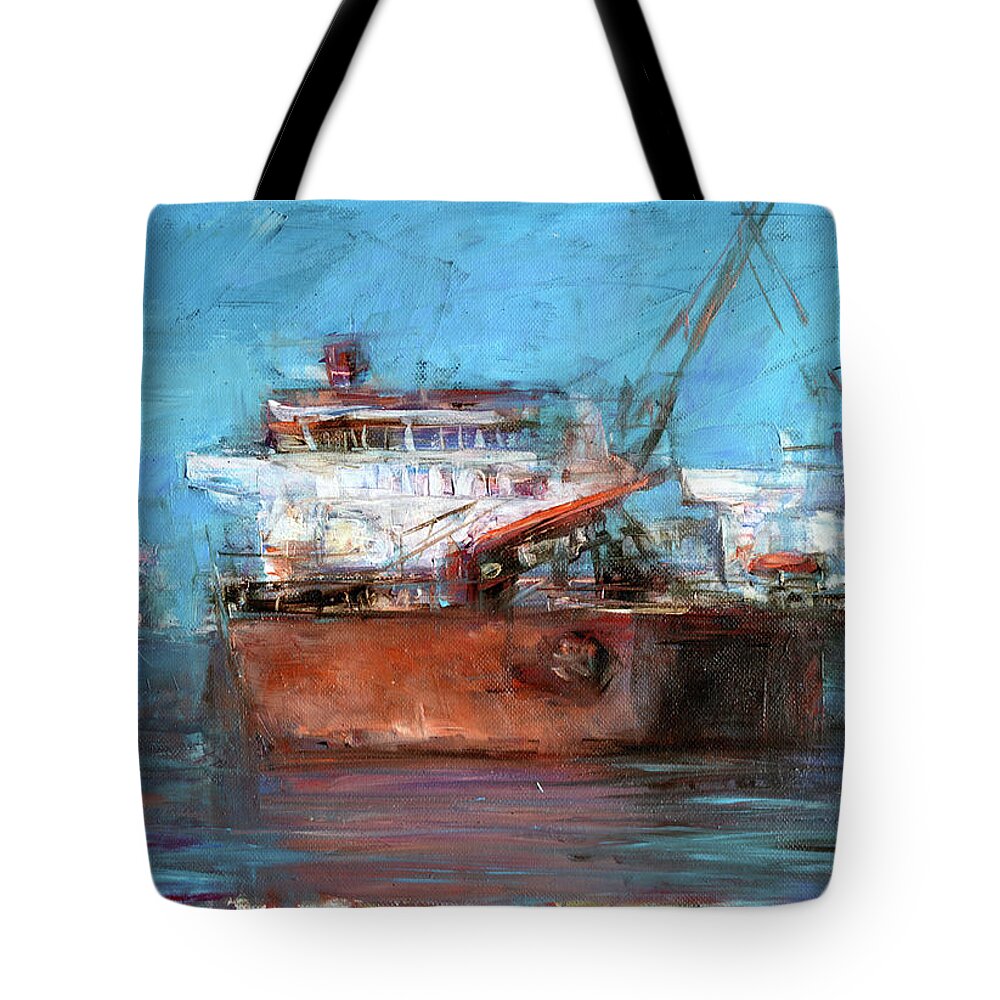The image depicts a square canvas tote bag, set against a plain white background with slight shadowing on the lower right side and bottom. The bag features two black handle straps emerging from the top, though their full length is cut off. The bag itself bears a painted design. The upper half of the painting depicts a clear blue sky with brush strokes that create a scratch-like texture. Below, a large watercraft, predominantly white with orange-red tones, sits in blue water. The paintwork on the bag is somewhat haphazard, creating a somewhat abstract representation of the scene. The reflection of the watercraft is seen in the water, although the water appears in greenish-gray hues rather than blue. The design is simplistic and takes up most of the bag's surface, enhancing the vessel's prominent presence.